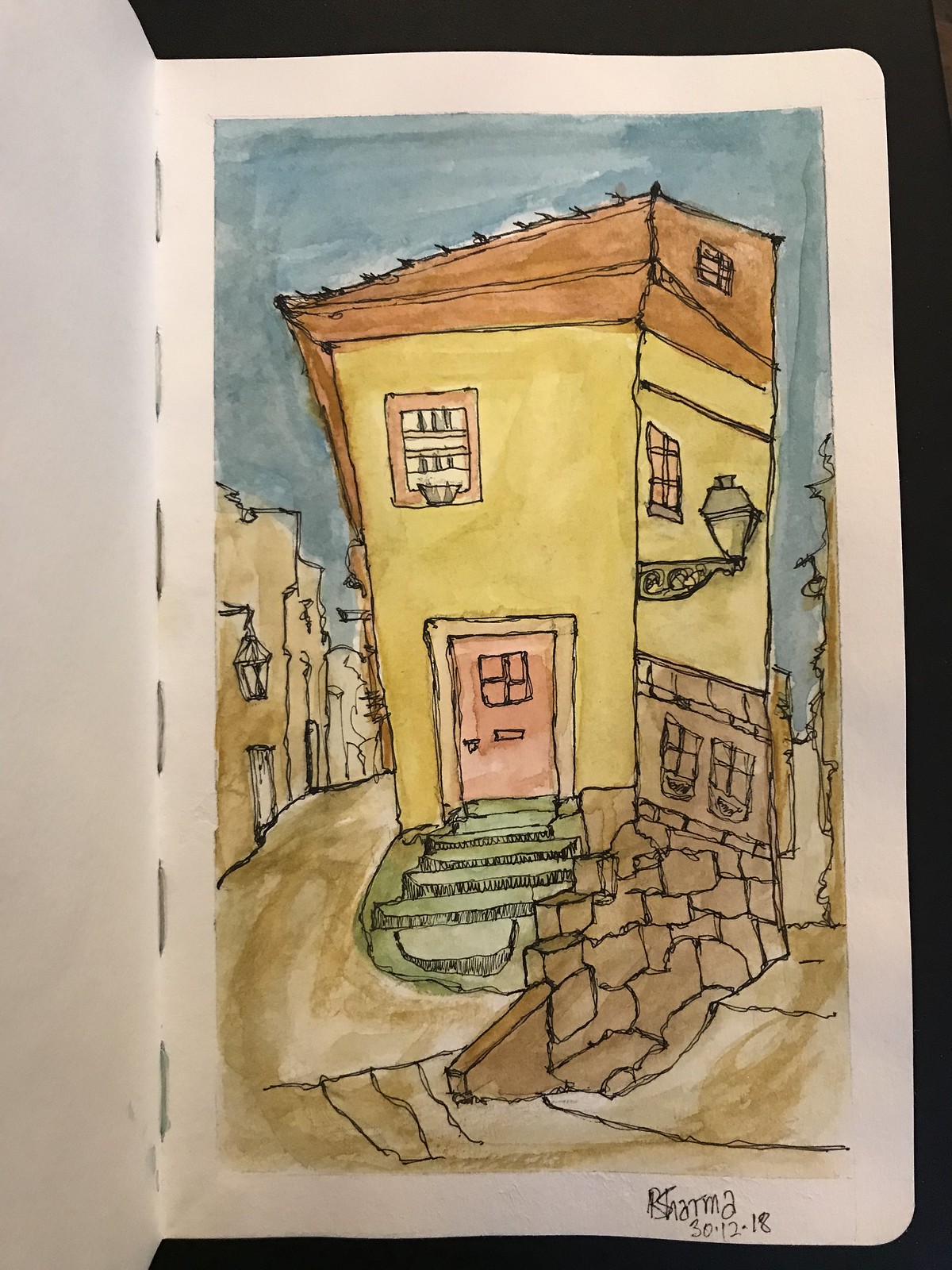The image depicts a detailed, stylized illustration of a European-style house created with watercolors on a slightly rounded, white piece of paper, folded on the left side. The yellow building is narrow, rectangular, and appears to be a few hundred years old, showing off a smooth, stucco-like exterior. It stands at least two stories tall, potentially three including an attic space. The roof is angled and brown, complementing the red front door accessed by green steps. An old-fashioned lamp post juts out from one side. The house is elevated on a rocky ledge with a curving road leading to similar-looking houses. The background features a blue sky and brown sidewalks. The artist's signature, "RSHARMA ARSHAMA DEDI 1218," is marked in black ink at the bottom right corner. The paper rests on a black surface, emphasizing the clean lines and detailed colors of the artwork.